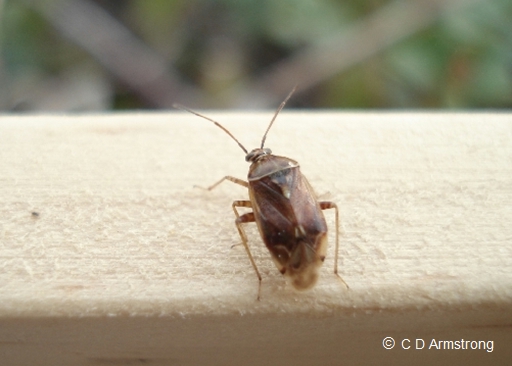In this well-lit daytime photograph credited to C.D. Armstrong in white text at the bottom right corner, a brown bug, possibly a cockroach, is standing upright on its back legs atop a beige surface. The surface looks like it could be a windowsill or a wooden ledge. The image is a striking close-up, with the bug prominently centered in the foreground. It displays six legs and two large antennae. Behind the bug, the background is artistically blurred, featuring muted tones of green, brown, and black, resembling foliage or leaves, which adds to the depth and focus on the insect.